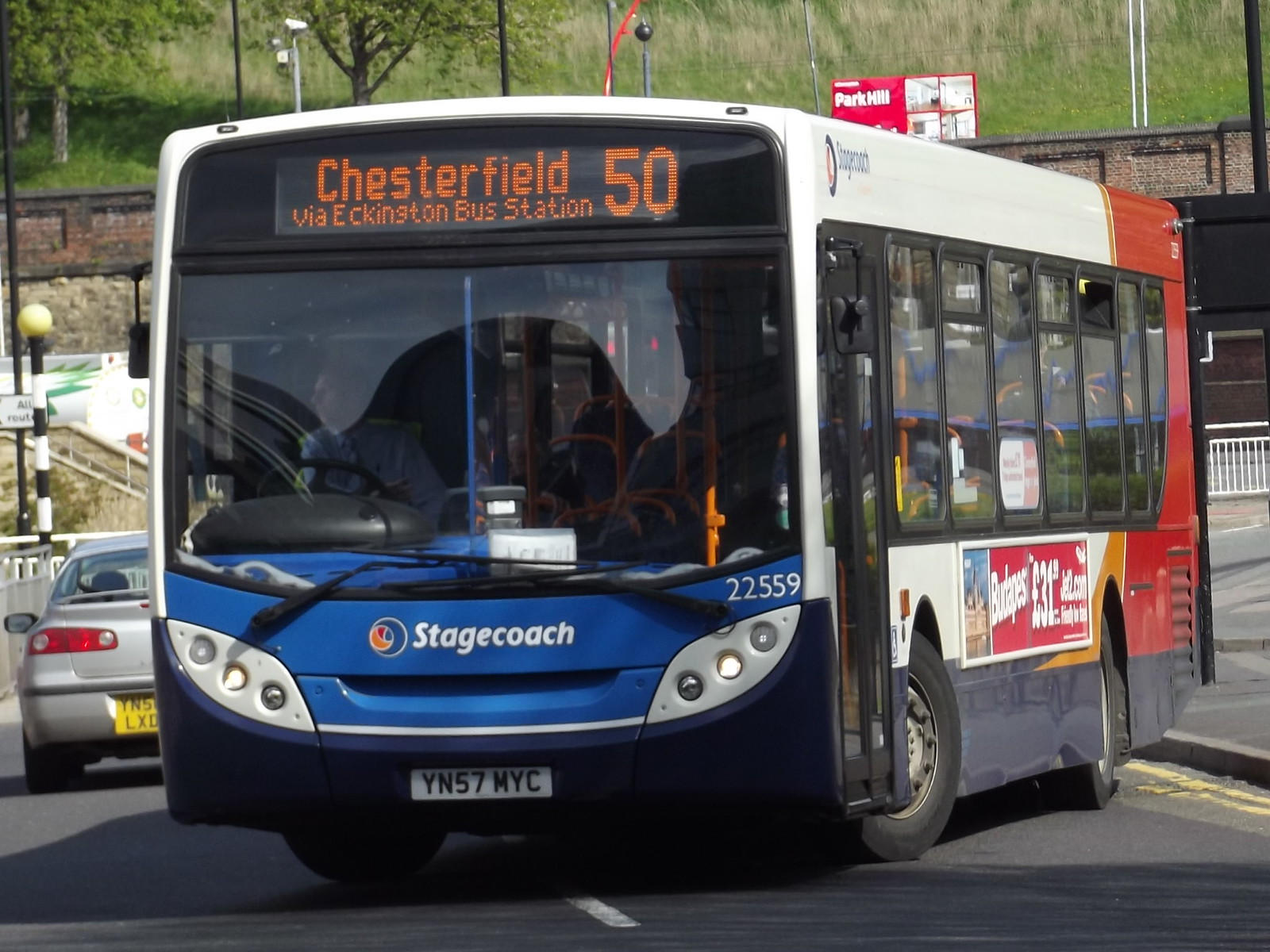The image depicts a Stagecoach bus just pulling out from a bus station, heading towards Chesterfield via Ekington bus station. The bus, numbered 50, has a large, prominent digital sign in orange letters at the top front façade. The bus features a distinctive color scheme with a white top, a red rear section, and a mostly blue front underneath the windshield adorned with the Stagecoach logo in white letters. The bus driver, a man, is visible through the large front windshield, diligently checking for traffic as he pulls out. The black bumper beneath the windshield is accompanied by a license plate reading YN57NYC. The side of the bus sports some advertising and a red banner. In the street beside the bus, there's a gray car with a yellow license plate moving in the opposite direction. The surrounding environment hints at an urban setting, with grass and trees visible in the background, partially obscured by a bridge and wall. The bus's position and the shadow on the street suggest it is daytime, enhancing the details of the bus and its surroundings.